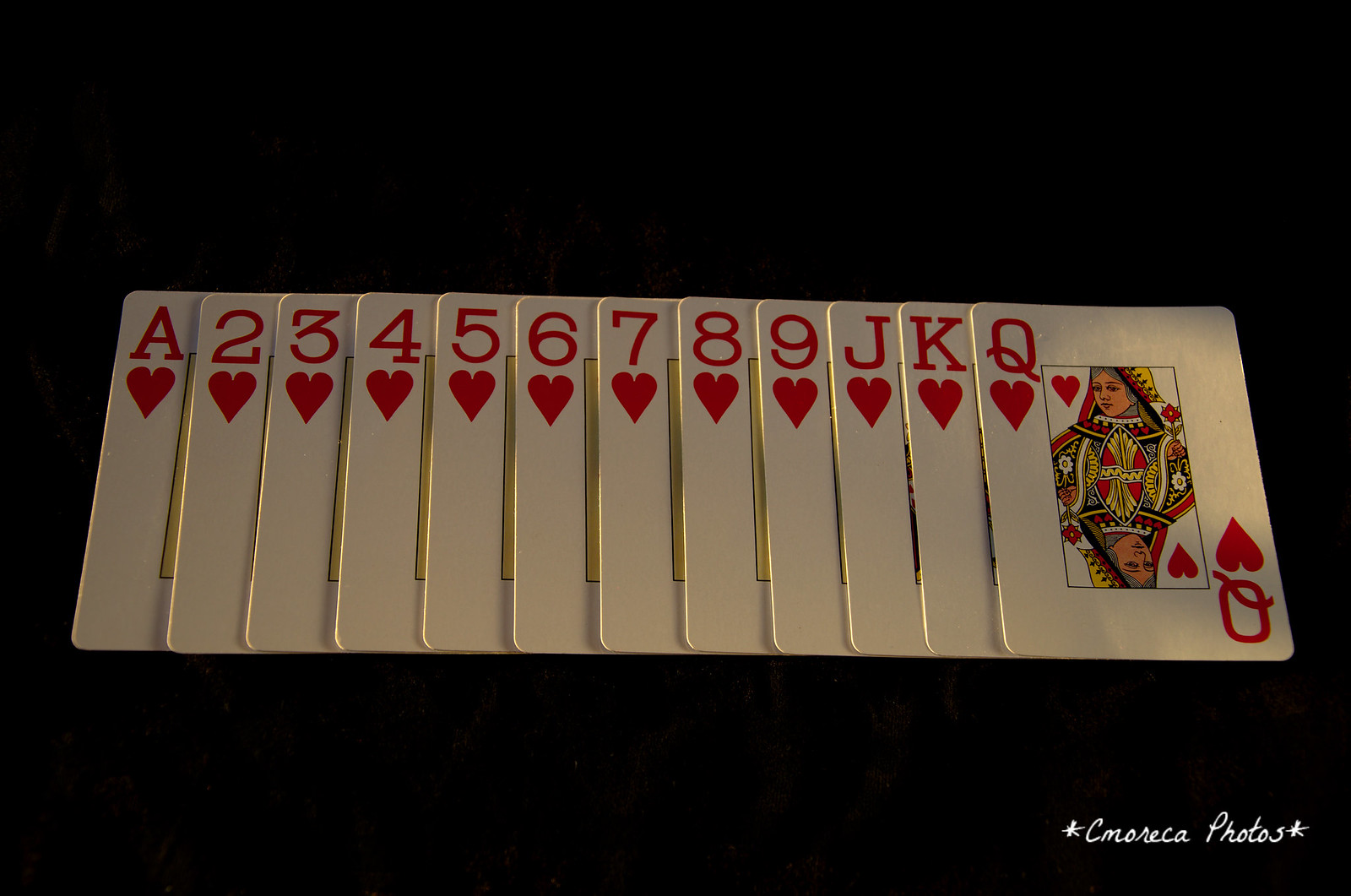The image features a stark black background with a series of playing cards laid out prominently in the foreground. At the bottom right of the image, there is a small graphic of a star followed by the text "C-M-O-R-E-C-A P-H-O-T-O-S" and then another star, suggesting it might be the signature or watermark of the photographer.

Focusing on the main content of the image, a sequence of playing cards, all of the heart suit, are arranged next to each other. Starting from the left, the sequence includes the Ace of Hearts, followed by the Two, Three, Four, Five, Six of Hearts. The alignment of these cards is slightly askew, not perfectly straight, but still clearly visible. The sequence continues with the Seven, Eight, and Nine of Hearts, skipping the Ten, and resumes with the Jack, King, and finally, the Queen of Hearts. The cards vary slightly in their positioning, with the face cards being particularly misaligned, further emphasizing the absence of the Ten of Hearts in the otherwise continuous suit sequence.